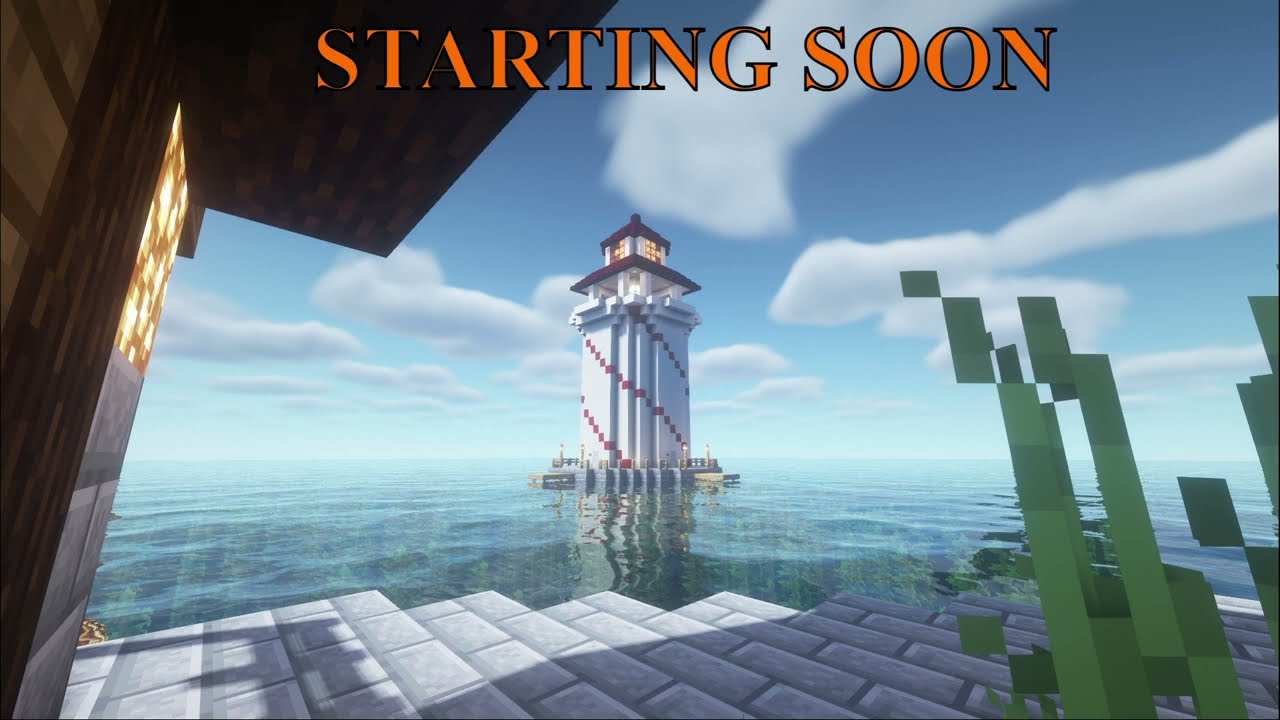The image depicts a clear blue daytime scene within a video game. Dominating the scene is a white lighthouse with red diagonal banners and a brown top standing on a large body of water, with its illuminated lantern at the top casting a yellow light. The lighthouse’s base is gray, and it features the bold orange capitalized text "STARTING SOON." To the left of the lighthouse, there's a brown building with an overhanging black roof, featuring windows with yellow, gold, and brown hues, and a brown door. Stone brick steps lead down to the water, where faint little waves can be observed. On the right-hand side, there are pixelated green rectangles of indeterminate objects. The sky above is a serene blue adorned with scattered white clouds.